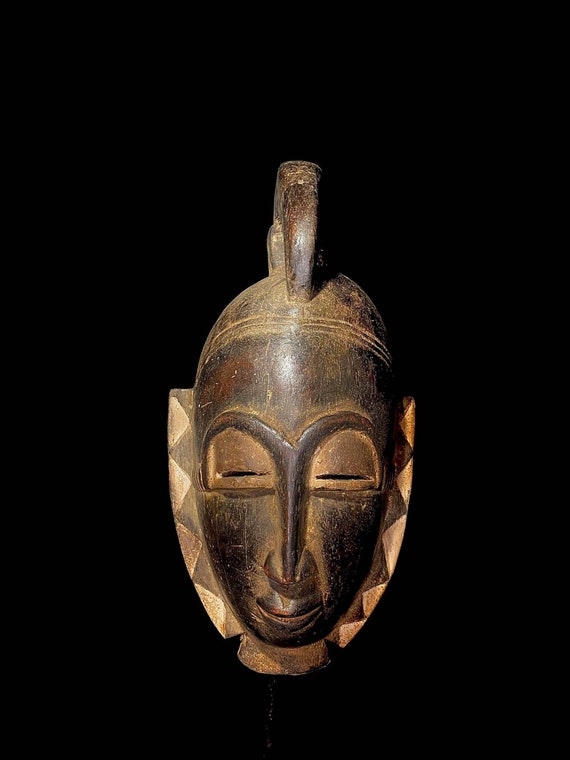This photograph depicts a detailed, antique tribal African mask set against a completely black background. The mask, which appears to be carved from polished wood and stone, exhibits a rich dark brown color with a hint of black. The face of the mask is oval or egg-shaped, and it features exaggerated facial elements. The eyes are represented by narrow slits under arched brows, while the nose is remarkably long and anchor-shaped. The mouth is small, contributing to the mask's serene, almost smiling expression. Additionally, the mask's forehead is prominent and is adorned with three horizontal lines. At the top, it boasts an elongated structure resembling a mohawk. Surrounding the face, from ear to ear and extending under the chin, is a distinctive diamond pattern in dark brown and white, possibly representing a decorative neckpiece or part of a helmet.